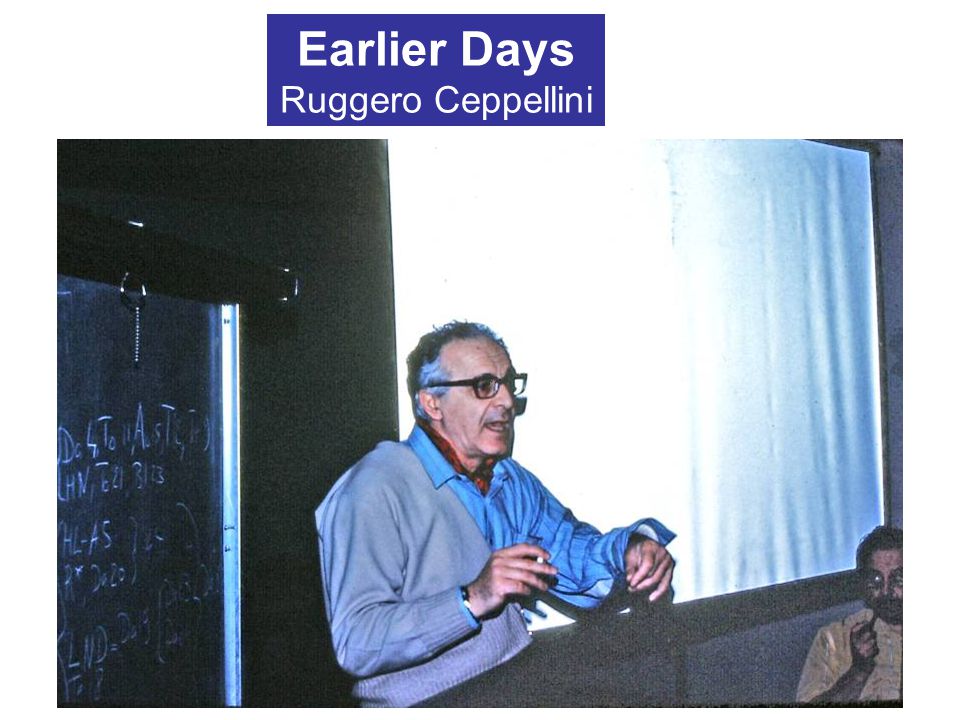The photograph depicts an older gentleman with a mix of gray and black hair, adorned in thick black-rimmed glasses. He's energetically lecturing, evidenced by his raised hands and open mouth, likely caught mid-explanation. The man is layered in clothing: a grey sweater over a blue dress shirt, and a red shirt peeking underneath. Chalk is clutched in his right hand as he stands centered in front of a chalkboard on his right, which has indecipherable text written in white chalk. Behind him is a white projector screen. To his left in the image, a seated man in a yellow shirt, sporting glasses and holding a smoking pipe, listens attentively. Above the scene is a blue rectangle with the white text, "Earlier days, Ruggiero Cepollini."